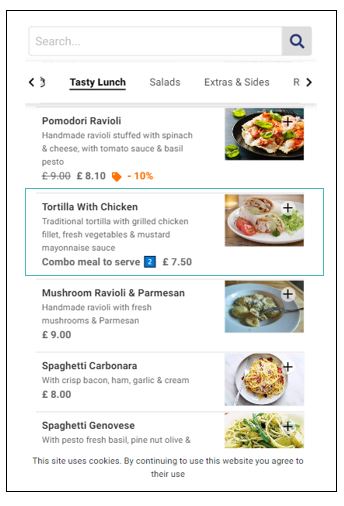This image showcases a screenshot of an online menu. At the very top of the menu, there is a search bar featuring a magnifying glass icon at its far end. Directly below the search bar, three tags are displayed: "Tasty Lunch" (bolded and underlined), "Salads," and "Extras and Sides."

The menu lists five different dishes:
1. **Pomodoro Ravioli** – Priced at £8.10, this dish is marked with a 10% discount.
2. **Tortilla with Chicken** – A combo meal serving two, priced at £7.50. The dish is highlighted in a box, and there is a plus icon at the top right corner of the dish's picture.
3. **Mushroom Ravioli Parmesan** – This dish is listed for £9.00.
4. **Spaghetti Carbonara** – Priced at £8.00.
5. **Spaghetti Genovese** – The price is not specified in the description.

Each menu item is formatted with the dish's name and a brief description on the left, followed by the price and any applicable discounts. The original price, when altered, is struck through. To the right of each item, a picture of the dish is displayed, featuring a plus sign at the top right corner.

At the very bottom of the menu, there's a notice stating: "This site uses cookies. By continuing to use this website, you agree to their use."